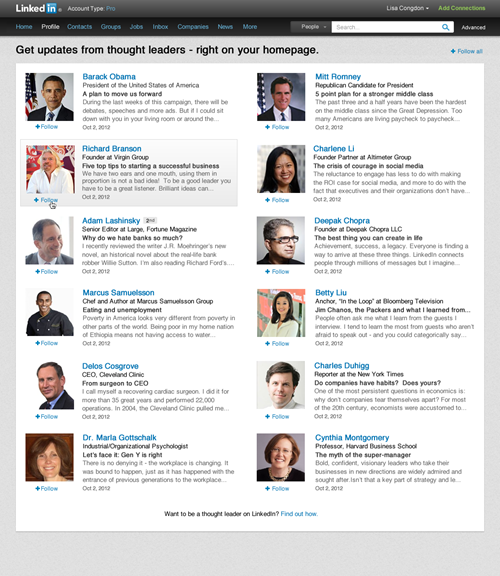The image features a gray background with a white rectangle centered within it. At the top of the white rectangle, spanning from left to right, is a black header containing the LinkedIn logo in white text on the left. On the right side of this black header, there is a search bar complete with a magnifying glass icon.

Below the black header, within the white rectangle, the text "Get updates from thought leaders right on your home page" is prominently displayed in black. The lower section of the white rectangle is dominated by two columns, each containing six photos of influential people along with short descriptive paragraphs beneath each photo, all against a white background.

In the left column, the featured thought leaders are:
1. Barack Obama
2. Richard Branson
3. Adam Lashinsky
4. Marcus Samuelsson
5. Delos Cosgrove
6. Dr. Maria Kotzschalk

In the right column, the featured thought leaders are:
1. Mitt Romney
2. Charlene Li
3. Deepak Chopra
4. Betty Lou
5. Charles Duhigg
6. Cynthia Montgomery

Each of these individuals has a brief paragraph underneath their name and photo, providing details about their background and contributions. The paragraphs are printed in a small font, making them difficult to read from a distance.